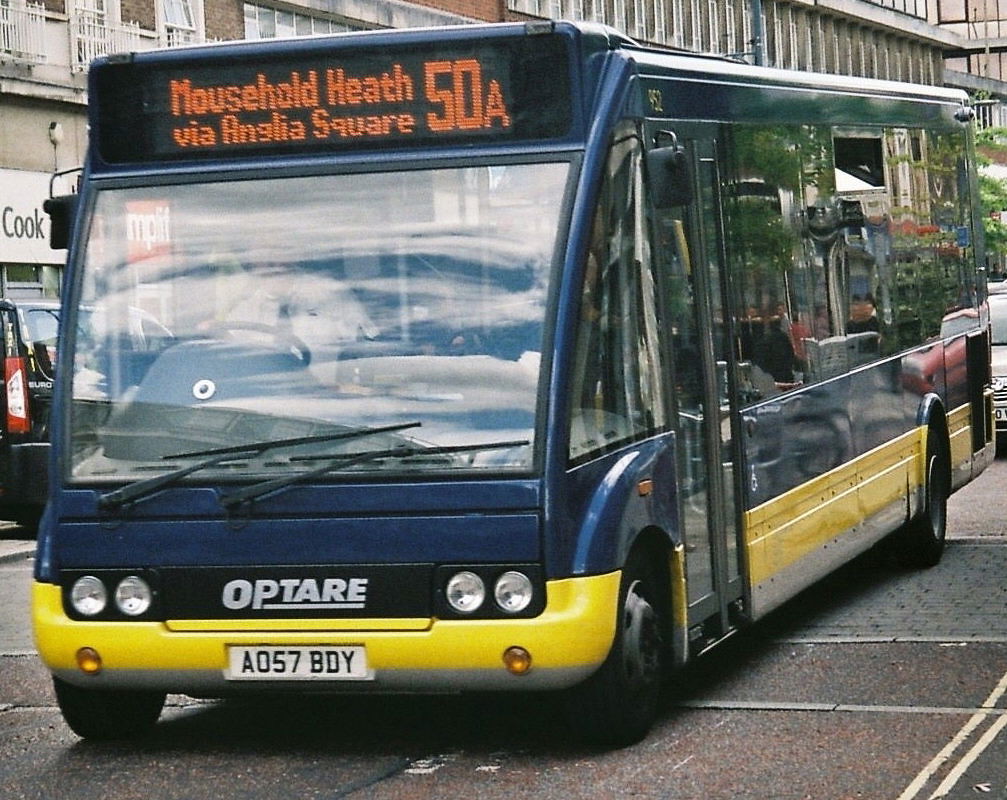This color photograph captures a large navy blue city transit bus with a distinctive yellow stripe around its lower quarter, prominently occupying the majority of the image. The bus, an Optare model, is in service and driving down a bustling city street. Central to the composition is the bus's clean and reflective front windscreen, mirroring a blue sky with scattered clouds. The LED sign above the driver, who is seated on the right side indicating a European setting, displays "Mousehold Heath via Anglia Square 50A" in bright orange text against a black backdrop. Beneath this sign, the license plate A057 BDY is clearly visible. In the background, urban architecture including a tall building and a partially visible store sign reading "Cook" in white text on black, frames the cityscape.